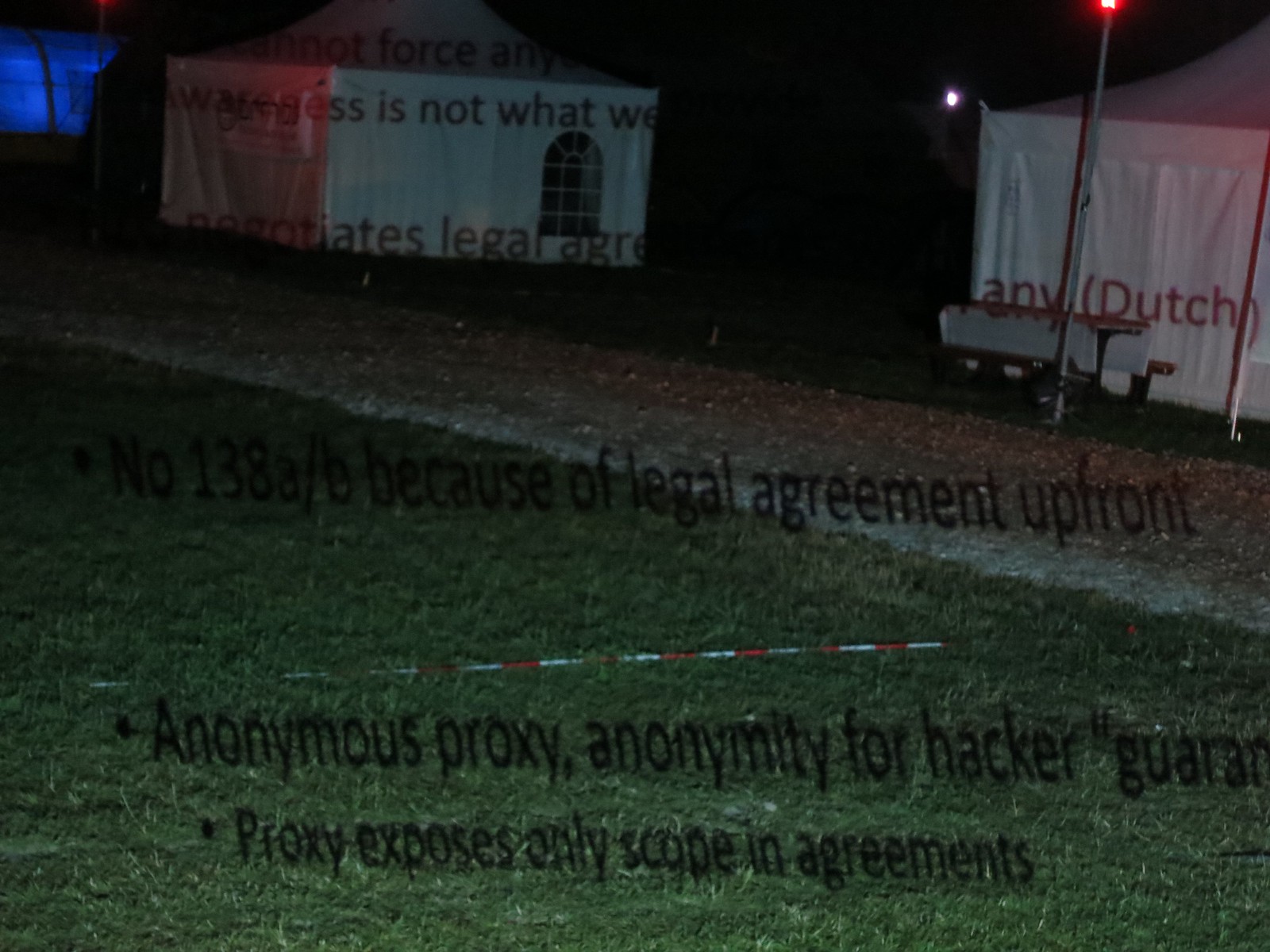This nighttime image features a dark grassy foreground and a winding white path, likely made of crushed stone, extending from the middle right to the upper left. In the background, there are a series of peculiar white tents shaped like houses, complete with faux plastic windows that mimic real ones. A striking red and white stick lies on the grass, alternating colors along its length, while in the top right corner, a silver pole with an intensely bright red light at its top stands out. Overlaid on this scene are various words and phrases: at the bottom center, it reads "bullet point, anonymous proxy, anonymity for hacker, gerun," with the incomplete phrase "proxy exposes only scope in agreements" beneath it. Additionally, towards the middle of the image, it states "bullet point, NO138AB, because of legal agreement up front." An isolated area of blue light is visible at the very upper left, providing a contrasting hue to the otherwise dark and mysterious setting.